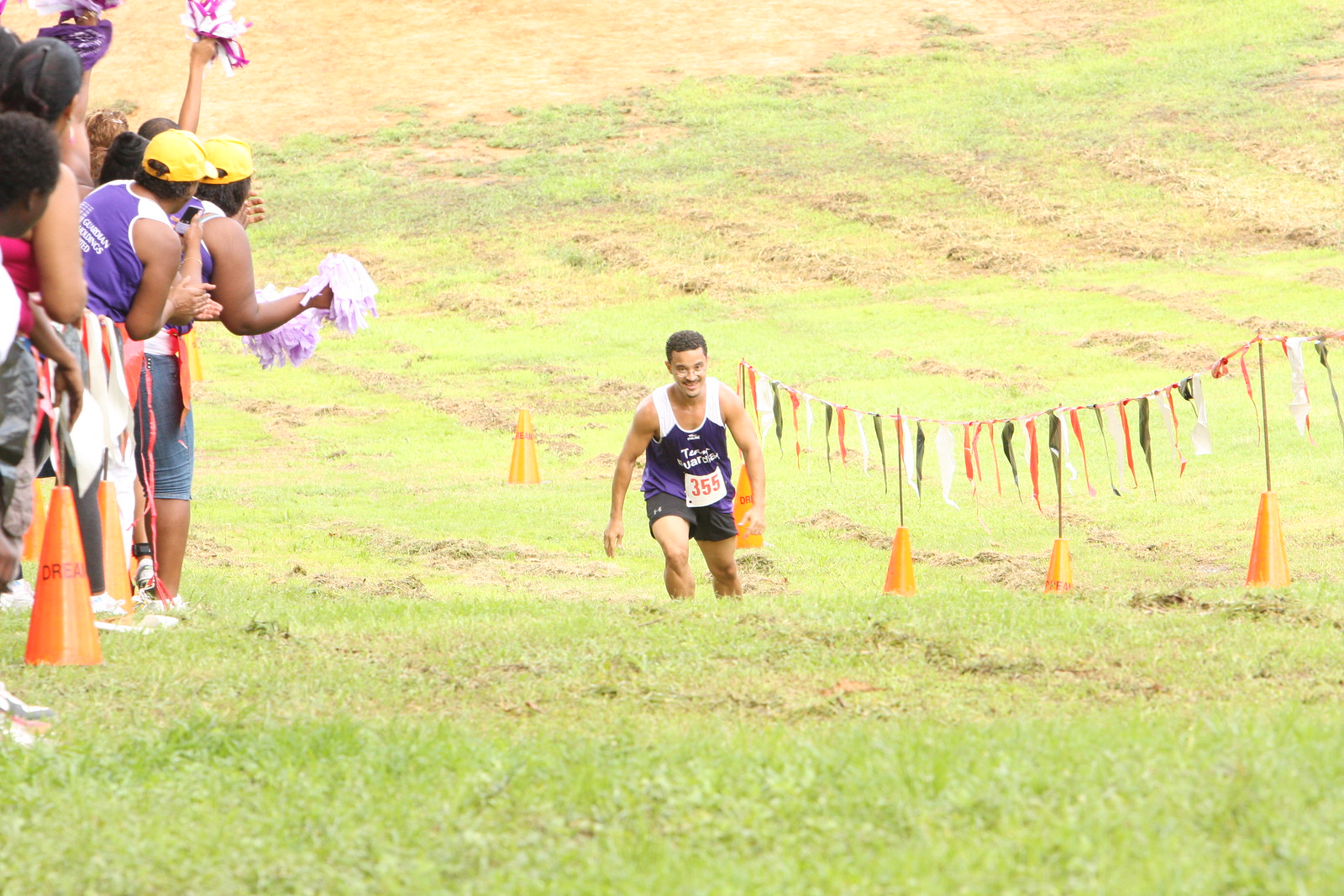In this vibrant outdoor photograph, the camera looks down a grassy hillside, partially dotted with clumps of dead, straw-like mowed grass. A runner, wearing black shorts and a blue sleeveless top with white shoulder straps, is captured mid-stride as he ascends the hill. Pinned to his vest is a red number 355, identifying him as a participant in what appears to be a long-distance marathon or cross-country race. The hillside is marked with orange cones running parallel to the path, some bearing metal poles adorned with red, white, and green triangle bunting flags. Along the left edge of the photograph, a group of enthusiastic spectators clad in casual attire, including yellow baseball caps and purple tank tops, cheer on the runner. Some of them wave purple pom-poms with streaming ribbons, adding to the festive atmosphere as they encourage the athlete on his uphill journey.